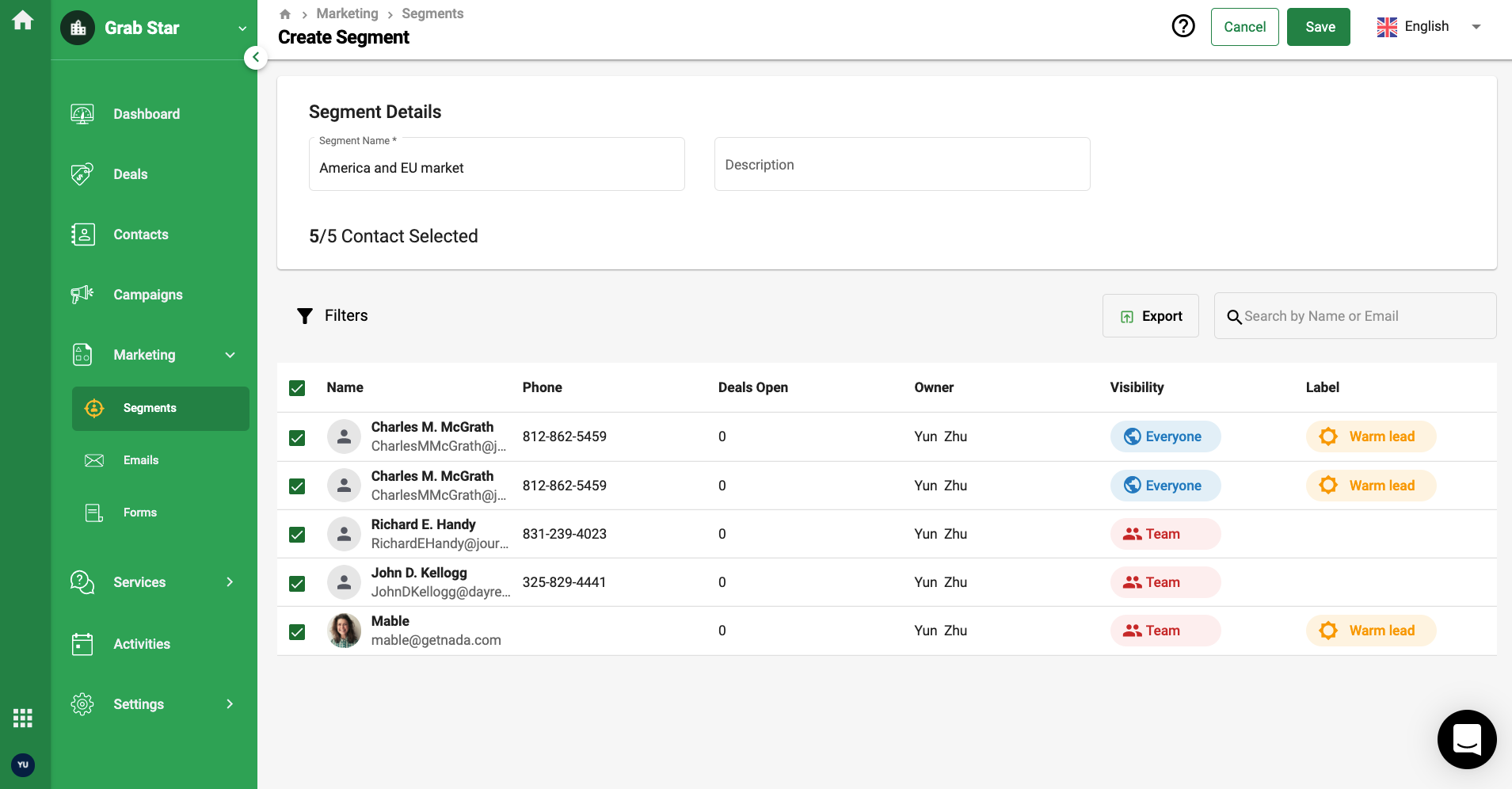The image depicts an ultra-wide computer screen displaying a detailed interface. On the left sidebar, the heading "Grab Star" is prominently shown, followed by a long, narrow green rectangular box. Below this, various navigational links are listed, including Dashboard, Deals, Contacts, Campaigns, Marketing, Segments, Emails, Fonts, Services, Forums, Activities, and Settings. The main screen is currently focused on "Segment Details" for marketing segments, highlighting data for the American and EU markets. It specifies that 5 out of 5 contacts are selected within this segment. The contacts listed include Charles McGrath (appearing twice), Richard Handy, John Kellogg, and Mabel. Each entry provides details such as phone numbers, open deals, owners, visibility, and labels, with Yun Zhu identified as the owner. Initially, it might seem related to Grab Taxis, a ride-hailing service similar to Uber in Southeast Asia, but the context confirms it is actually focused on marketing segment details.